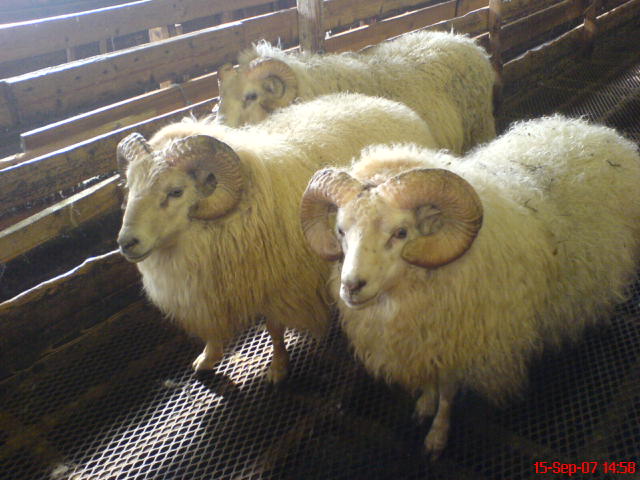This color photograph, taken inside a barn or wooden trailer on September 15, 2007, at 2:58 PM, captures the scene of three wild rams, identifiable by their large, curved horns. The rams, which have scruffy, cream-colored wool tangled with dirt, leaves, and hay, are standing on a metal grate that serves as the flooring. The two rams in the front are looking directly at the camera, while the third stands slightly behind them. A wooden fence, approximately four feet high, forms a barrier in the background to keep the rams enclosed within the pen, contributing to the rustic and earthy setting of the image.